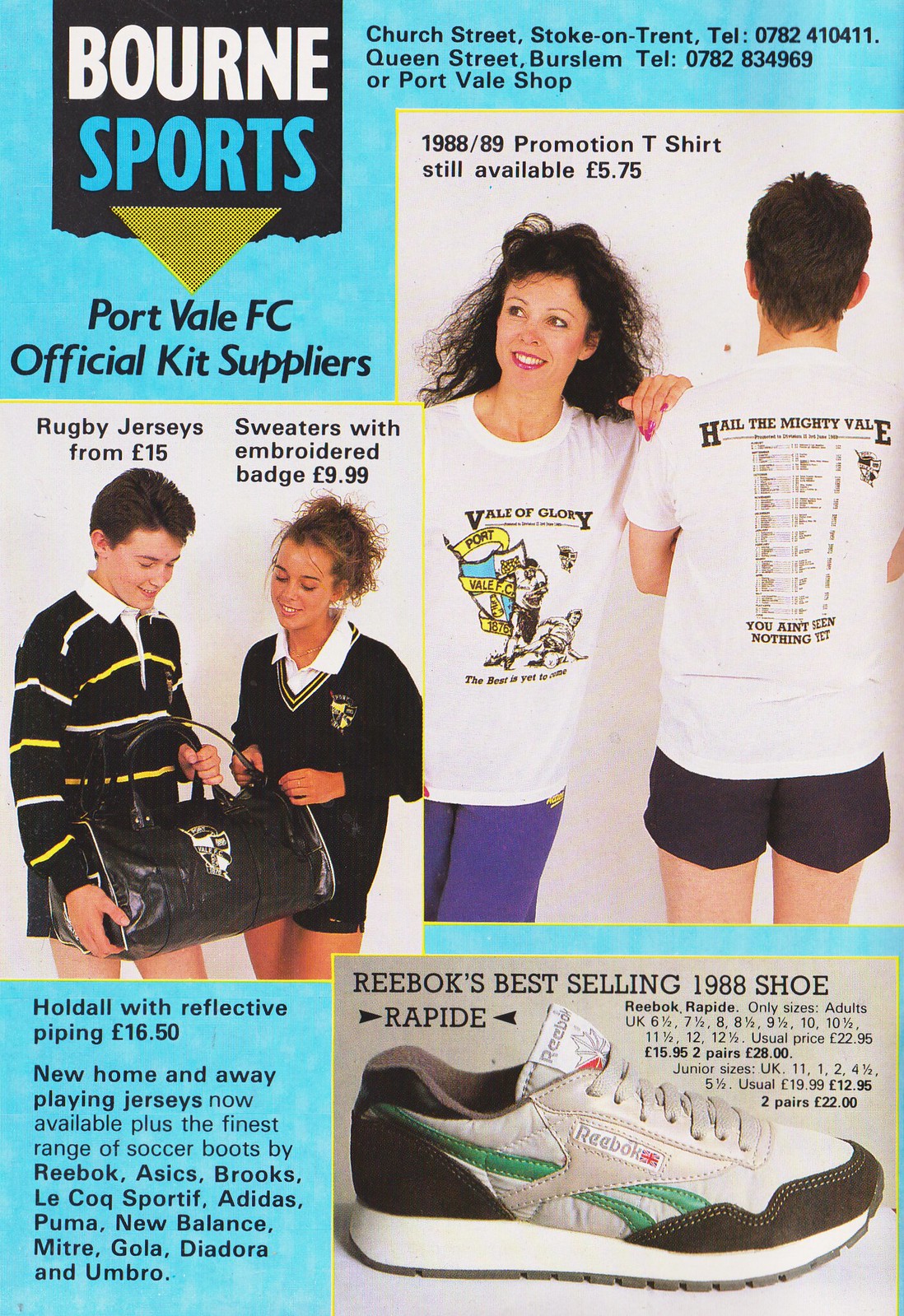The advertisement page from a magazine features a detailed layout for Bourne Sports, prominently displaying their UK locations at Church Street, Stoke-on-Trent, and Queen Street, Burslem, complete with telephone numbers 0782410411 and 0782834969 respectively. Central to the ad is the announcement that Bourne Sports is the official kit supplier for Port Vale FC, showcasing their new home and away playing jerseys. The ad highlights a range of products including rugby jerseys starting from £15 and sweaters embroidered with the club badge from £9.99. There's also a promotion for 1988-89 season t-shirts priced at £5.75. At the bottom of the page, there are advertisements for Reebok's best-selling 1988 Rapide shoe, available in UK sizes and various prices from £22 to £28. In addition, a hold-all with reflective piping is listed for £16.50. The brands featured include prestigious names such as Reebok, Isaac, Brooks, LeCog Sportif, Adidas, Puma, New Balance, Meter, Gola, Deodora, and Umbro. The visual includes a woman and a boy modeling the clothes, with text primarily in blue and black, creating a vibrant, yet organized, presentation.